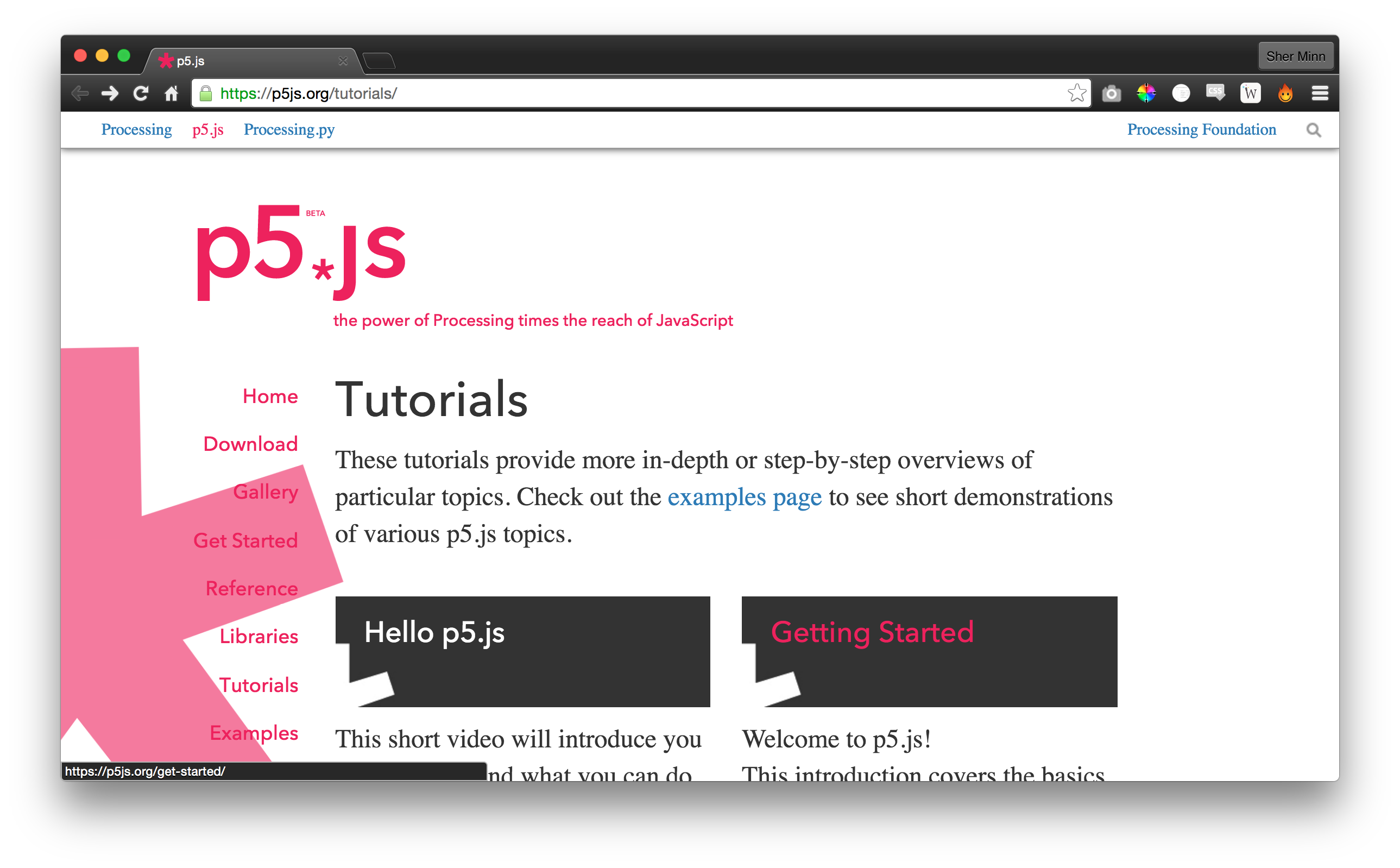The web page presented is the P5.js homepage, featuring a black-themed navigation bar at the top with white text showcasing main sections: "P5 Star JS," "Tutorials," "Home," "Download," "Gallery," "Get Started," "Reference," "Libraries," and "Examples," with some repetitions of "Tutorials." Below, a white section with black text outlines the offerings in tutorials, highlighting step-by-step guides and overviews on specific topics. The "Examples" page is emphasized with blue letters. Visual elements include a black square with "Hello P5.js" written in white letters and another with "Getting Started" in pink letters. A short introductory video is also featured, titled "Welcome to P5.js," which promises to cover the basics of the platform. The introductory message "P5.js. Welcome." is repeated three times dynamically across the interface.